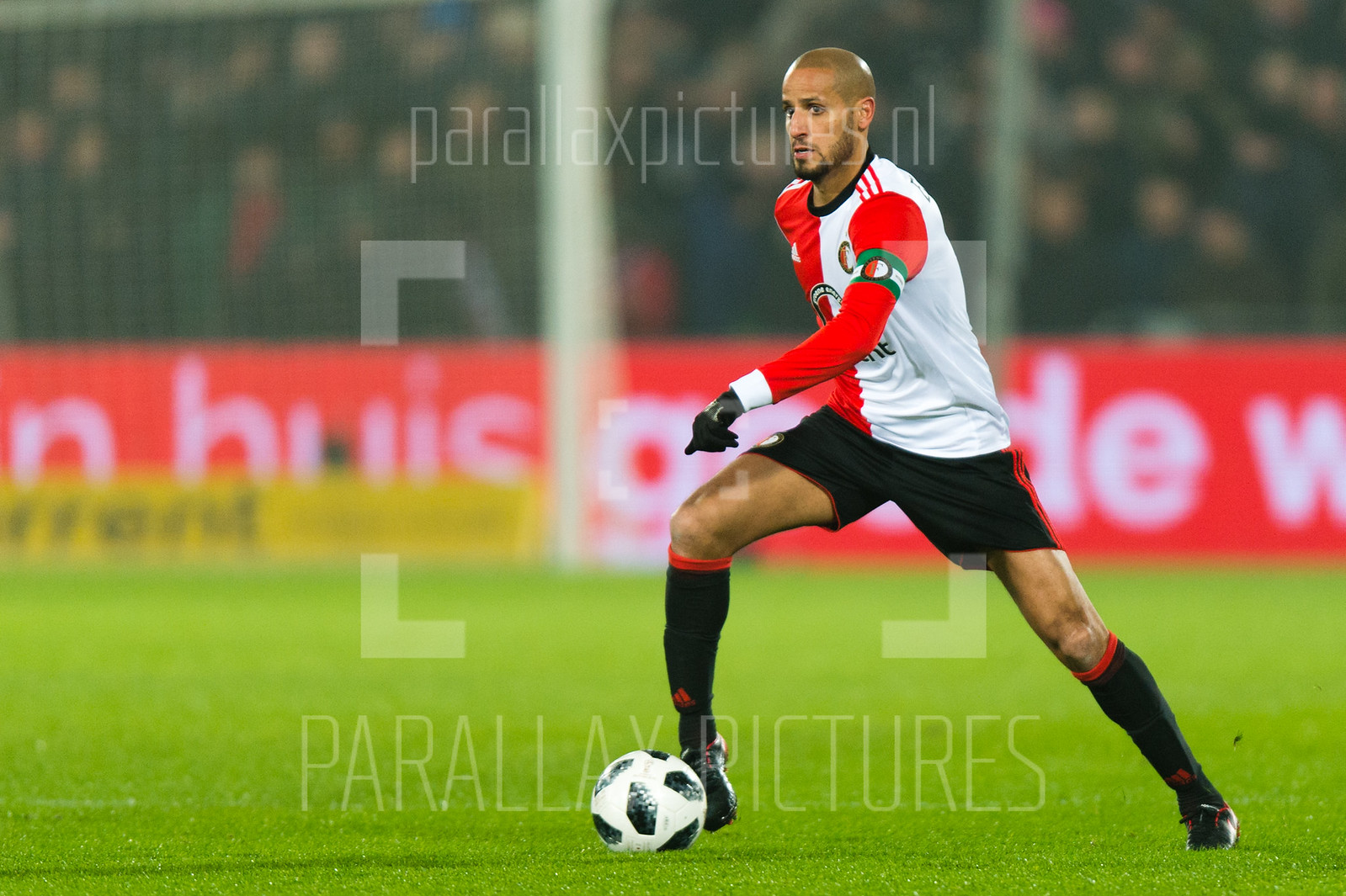This image, from Parallels Pictures, features a dynamic scene of a soccer player in action on a natural grass soccer field. The athlete, dressed in black shorts with red accents, black socks, black shoes, and a red and white long-sleeve jersey, appears intensely focused as he prepares to kick a classic black-and-white soccer ball. His head is shaved, revealing a hint of black hair, and he sports a noticeable beard, looking off to the right while running. His left arm extends forward, suggesting his swift movement across the field.

The photograph captures a crowded, albeit blurry, stadium backdrop, with indistinct figures of spectators filling the stands. A red banner is visible, likely bearing some form of advertisement. The image, framed within a viewfinder square and marked with a watermark "parallaxpictures.nl" at both the top and bottom, emphasizes the player as the focal point, with the background intentionally left out of focus to highlight his movement and the imminent action of kicking the ball.